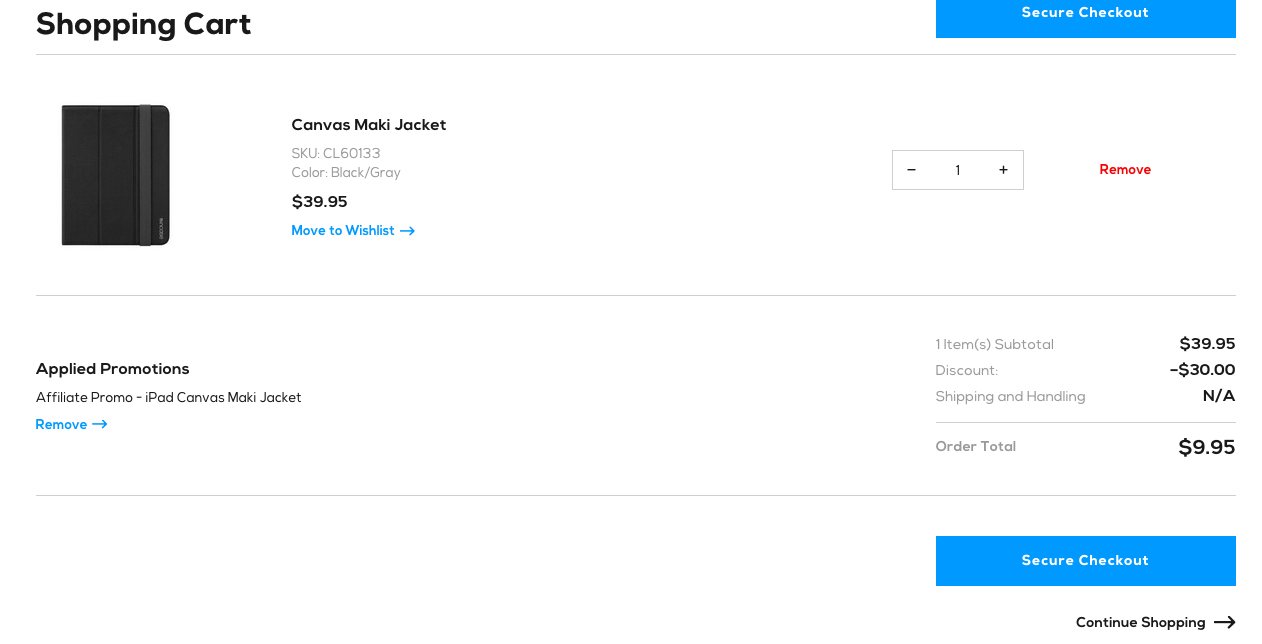The webpage displays a shopping cart interface. At the top, the heading "Shopping Cart" is prominently displayed. Below the heading, there is a blue "Secure Checkout" button. The cart contains an image of a small black-gray piece of material, identified as a "Canvas Maki Jacket." The jacket is listed as being black/gray in color and has a price of $39.95.

There is an option to move the item to the wishlist, highlighted in blue. The quantity for the item is set to one. Additionally, there is a red "Remove" button for the item.

Below the item details, in a section labeled "Applied Promotions," there is an entry for an "Affiliate Promo" specifically for the "iPad Canvas Maki Jacket." This section includes a blue "Remove" button and lists one item with a subtotal of $39.95. A discount applied to the cart deducts $30 from the total price. The section for "Shipping and Handling" states "Not Applicable."

The order total is displayed as $9.95. Most of the text on the page is in black or gray. There is another blue "Secure Checkout" button, as well as a "Continue Shopping" button in black, featuring an arrow pointing to the right. The entire webpage has a clean, white background.